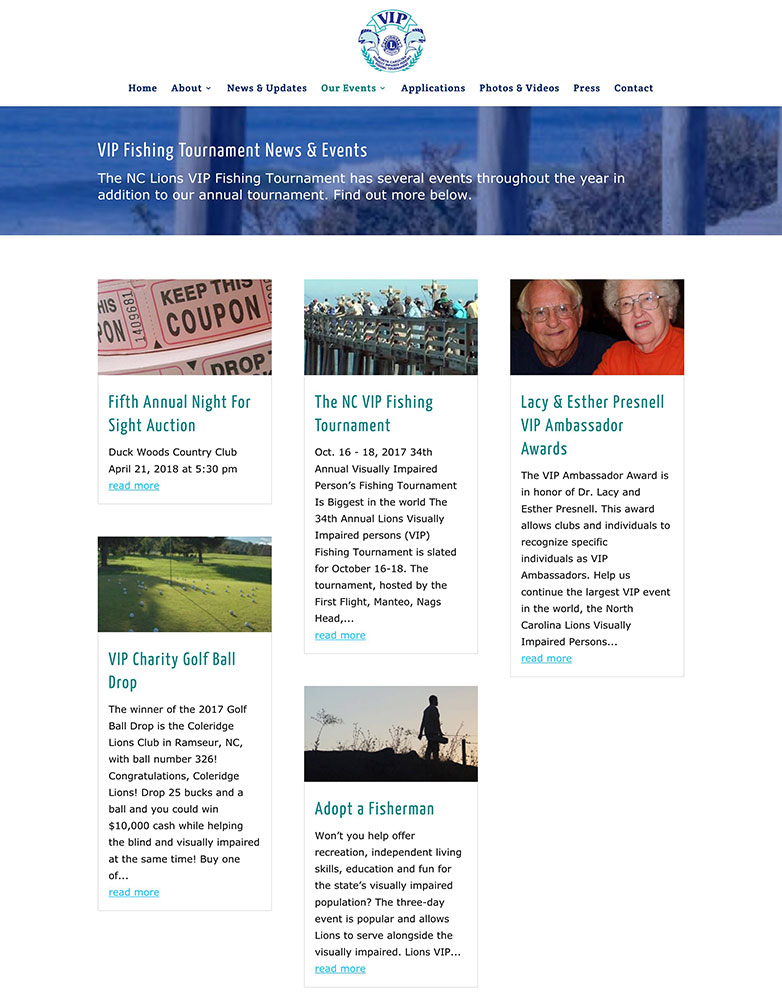The image depicts a professional government website with a clean and organized layout. At the top center of the page, the acronym "VIP" is prominently displayed, accompanied by a monogram featuring a stylized letter "L" and some unreadable text beneath it. 

The navigation bar below this header includes menu options such as Home, About, News and Updates, Our Events, Applications, Photos and Videos, Press, and Contact, all aligned towards the left side. Directly beneath this menu is a horizontal banner image illustrating the underside of a pier, with visible wooden supports. The banner text announces the "VIP Fishing Tournament" and categorizes it under "News and Events."

The main content area is divided into various sections featuring different events and news updates, each accompanied by relevant media images. On the left, the first article headline reads "Fifth Annual Night for a Site Auction," which includes a picture of coupons. Below that, another article titled "VIP Charity Golf Ball Drop" displays a media image of a golf course, followed by related event information.

To the right, the focus shifts to the "NC VIP Fishing Tournament," accompanied by a photograph of people standing on a pier and reading a comprehensive paragraph about the event. Subsequent articles include "Adopt a Fisherman" and "Lacey and Esther Presnell VIP Ambassador Awards," both featuring corresponding images. Each article concludes with a "Read More" link positioned at the bottom left, inviting viewers to access further details.